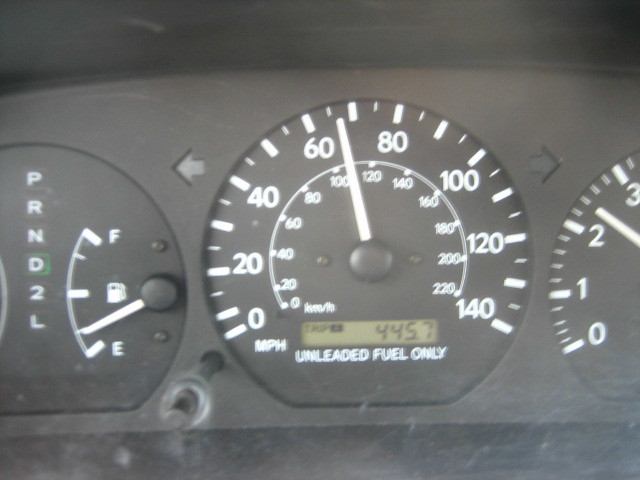The photo captures a detailed view of a car's black dashboard, featuring three central dials and various indicators. Dominating the center is a speedometer with white lettering on a black background, ranging from 0 to 140 MPH. The speedometer's markings increase in increments of 20, with smaller tick marks in between. The long white needle currently hovers slightly above the 65 MPH mark. Just below this needle is a small, rectangular LCD screen that reads 445.7 miles, accompanied by the text "unleaded fuel only."

To the left of the speedometer is a fuel gauge, indicating the tank is approximately one-quarter full. The gauge has four slash marks with an 'E' at the bottom and an 'F' at the top. Adjacent to the fuel gauge, a vertical column of letters, "PRND2L," shows that the car is in drive, indicated by a green-highlighted 'D.'

On the right side of the speedometer, partially visible, is another dial with a hand positioned between the 2 and 3 marks. This detailed setup illustrates the vehicle’s operational status, speed, fuel level, and gear, providing all necessary information at a glance.